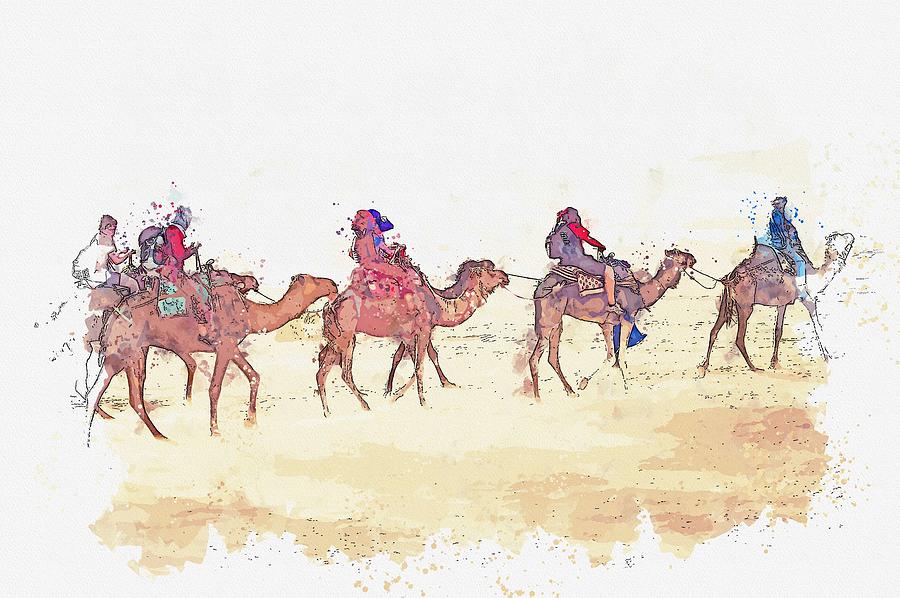The image is a digitally photographed piece of art, depicting an impressionist drawing of five brown camels traveling through a desert. The camels are moving from the left side of the image to the right, seemingly engaged in heavy labor as each camel carries a rider. The primary colors in the artwork are white and brown, with accents of blue, red, pink, and teal. The desert appears to be whipped by a sandstorm, suggested by the significant presence of white in the image, which may represent swirling sand. The riders on the camels are not as detailed as the animals themselves, with specific individuals wearing distinguishable clothing: the lead rider in blue, the second in red sleeves, the third in a white cap, and the last two riders in a red shirt and a white shirt respectively. The camels and figures are outlined in black, enhancing the abstract and impressionist style of the art. The ground beneath the camels is a light-colored sand, devoid of any sky or other background features.